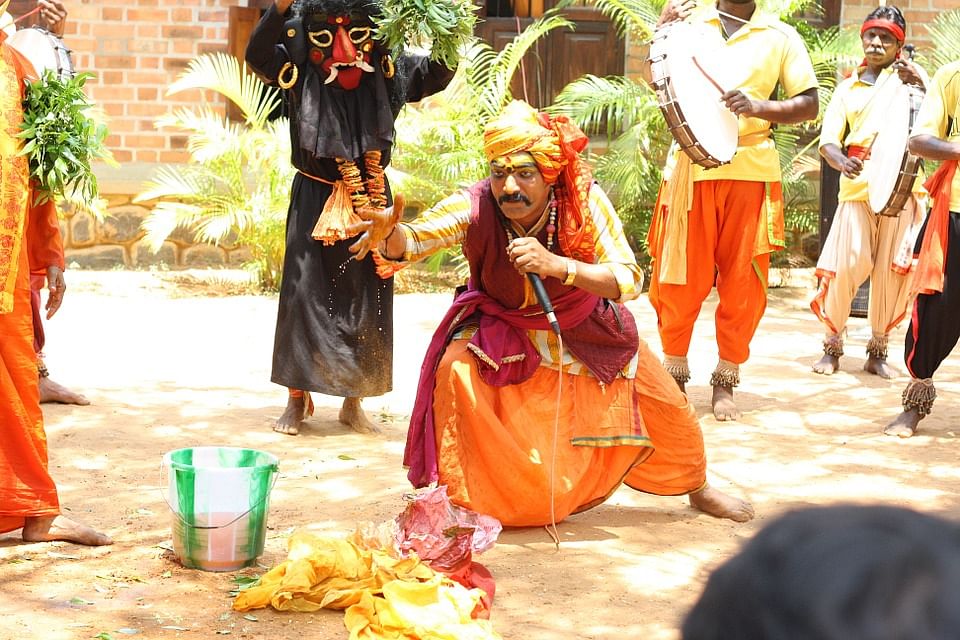This travel photograph, likely taken in India, captures a vibrant cultural scene centered around a man who appears to be performing some type of ritual or musical act. The man, possibly a shaman, is crouched down in the middle of the image wearing traditional Indian attire: bright orange pants, a long red scarf, and a yellow and orange turban. He is barefoot and holds a microphone in one hand while extending his other arm outward as if casting a spell or engaging in a ritualistic performance. The man has a mustache, some bees hovering around him, and something tied around his brow. Surrounding him are several individuals also dressed in colorful garments such as bright orange, yellow, and red robes, pants, and shirts. Some of these participants are playing large drum-like instruments, and one man is notably wearing a black garment and an ugly mask, possibly depicting a monster or demon. In front of the central figure, there are brightly colored cloths in yellow and red, and a white and green bucket whose contents are unknown. The background shows some plants, and the scene is brilliantly lit by the sun, indicating a bright, clear day. The overall ambiance suggests a lively and possibly religious or cultural ceremony.